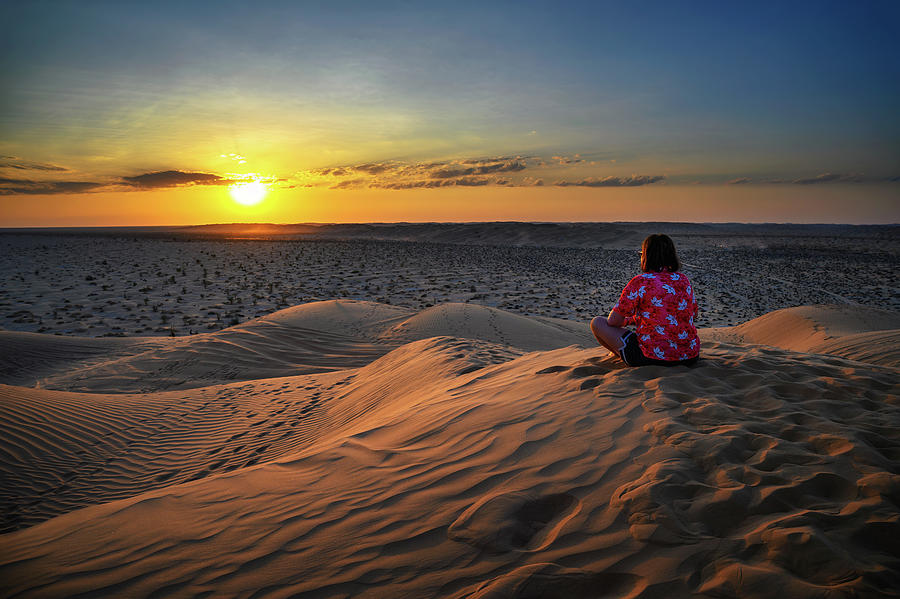In this artistic photograph, a woman sits cross-legged on the sandy dunes of an expansive desert, engrossed in the serene beauty of the setting sun. She wears a vibrant red shirt adorned with white flowers and dark shorts, with sunglasses resting on her short brown hair. Facing away from the camera and towards the breathtaking horizon, she contemplates the vast landscape, her figure silhouetted against the golden and bronze hues of the sunset.

The desert is alive with textures and patterns: the sand dunes exhibiting footprints and wind-shaped marks, while dried plant life punctuates the scene, adding a rugged beauty to the otherwise smooth terrain. The sky above features wispy cirrus clouds, enhancing the romantic lighting that bathes the entire landscape in a soft, warm glow. Shadows play across the sand, casting intricate designs that reflect the tranquil yet profound atmosphere of this moment.